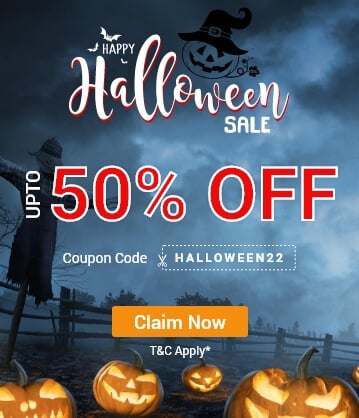The image features a festive "Happy Halloween Sale" announcement, prominently showcasing a discount of up to 50% off. To redeem the offer, shoppers can use the coupon code HALLOWEEN22. A note indicates that terms and conditions apply. The background of the image is a blend of grey, red, and pink hues, creating a spooky yet vibrant atmosphere. Scattered around the scene are intricately carved pumpkins, painted with a palette of orange, yellow, white, and black watercolors, adding a touch of traditional Halloween charm. To the left, a whimsical scarecrow stands amidst dark, ominous clouds, enhancing the eerie, otherworldly vibe of the promotion.